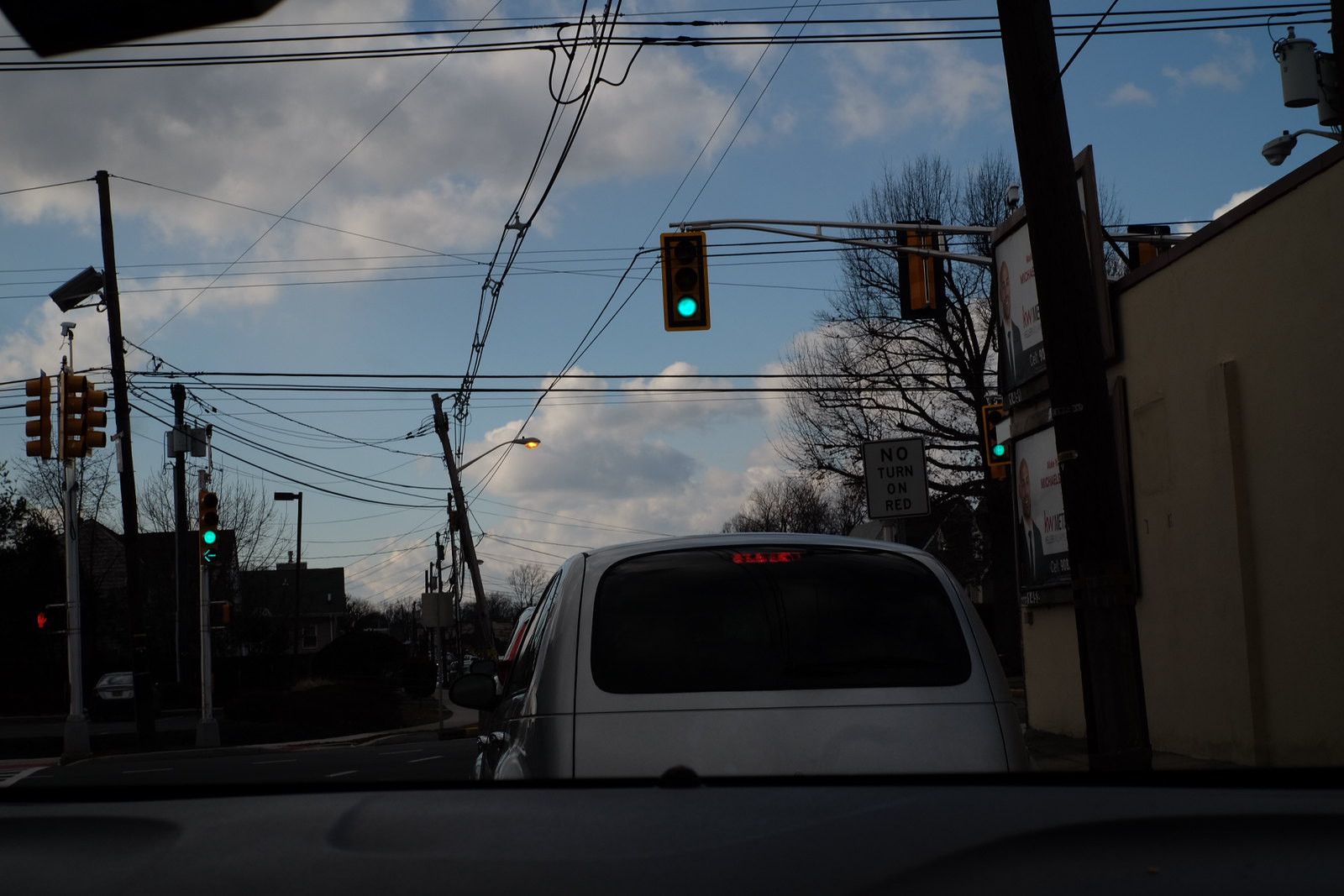This photograph, captured from a dashboard camera in a car paused at an intersection, depicts a late afternoon traffic scene. The dashboard, featuring gray with indented design details, is visible at the bottom edge of the image. Directly in front, a silver PT Cruiser-like vehicle with a distinctly black rear-view mirror and flat rear end is seen with its brake lights illuminated. Above this vehicle, the traffic light has just turned green, signaling the resumption of movement.

To the right, a prominent sign reads "No Turn on Red," situated above a brown building adorned with two billboards, each displaying a different person, possibly for a service or advertisement. Further right is a red pedestrian stop signal. The left side of the image reveals more traffic lights and shadows of distant apartment buildings or homes. 

The intersection is heavily laden with brown wooden utility poles and a complex network of power lines crisscrossing both horizontally and vertically across the scene. Bare-branched trees also dot the background. The sky is a bright blue with patches of gray and white clouds, suggesting a clear but not entirely cloudless day, perfect for travel.